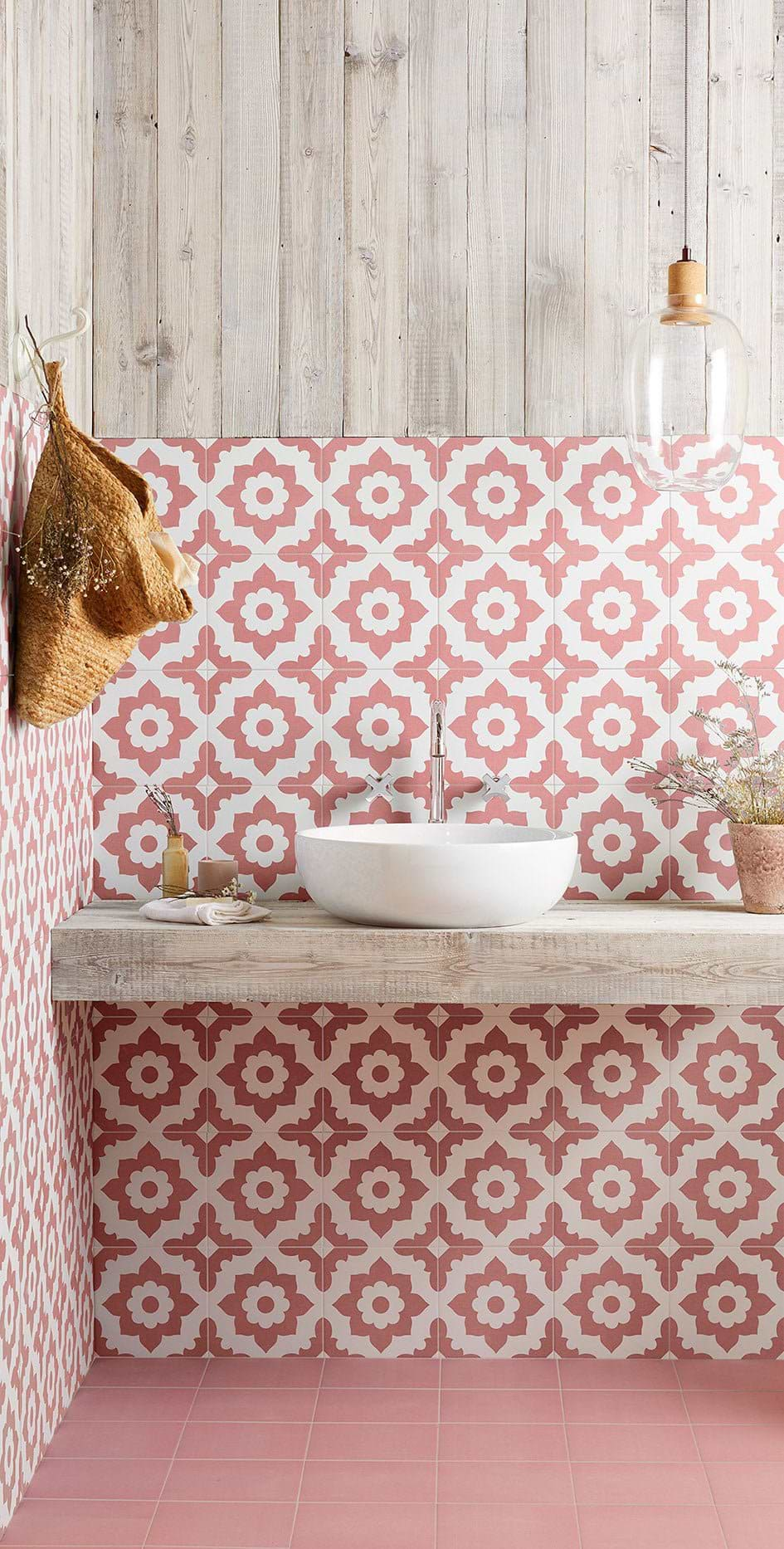The image showcases a quaint and visually intriguing corner of what appears to be a bathroom or vanity area, styled in a blend of boho chic and rustic. The walls are paneled with light gray, almost blonde wood, and the bottom two-thirds are adorned with a pink and white geometric design, possibly achieved through tiling or wallpapering. A substantial horizontal gray plank separates these two sections. Sitting atop this plank is a white, handcrafted-looking bowl sink featuring a silver faucet, suggestive of flowing water.

To the right of the sink is a flower pot brimming with wildflowers, adding a touch of nature to the scene. On the left is a rattan bag, seemingly filled with flowers, hanging from the wood-paneled wall. Beside the basin, a washcloth is neatly folded, while adjacent, there is a bottle that perhaps contains oil or another liquid. The floor below mirrors the wall's color scheme, adorned with solid pink tiles that give the space a cohesive and vibrant look.

Overhead, a light fixture with a clear glass globe dangles, casting a warm, ambient glow over the sink area. The eclectic mix of elements, from the clear glass light fixture and wooden panels to the pink-tiled floor and floral accents, creates a charming and cozy aesthetic that evokes a serene, laid-back atmosphere.